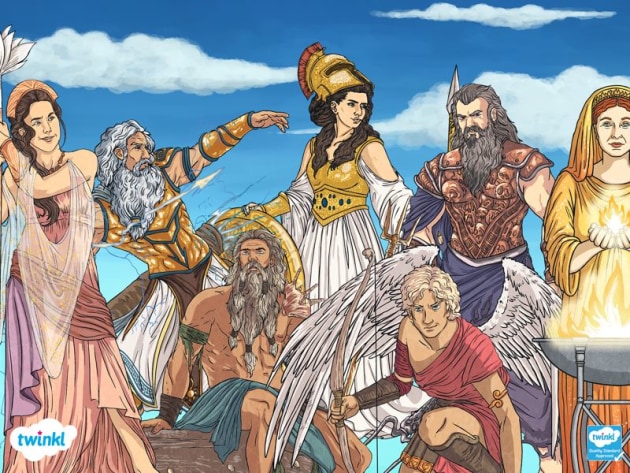The image is a detailed, colorful illustration reminiscent of Greek mythology, created by an artist associated with a brand called Twinkle, as shown by its turquoise logo with a white cloud in the bottom corners. The artwork features seven characters styled as Greek gods in a comic book fashion. Central figures include a bearded man with a white beard resembling Zeus, holding a lightning bolt, and another figure with blonde hair and white angel wings, holding a bow and arrow, resembling Hermes. A woman in a gold gown and headdress holds a flame, suggesting she might be Hestia or another goddess associated with fire. There is also a rugged, armored man who could be Ares. Other female figures include one in a helmet, hinting at Athena, and another adorned with a crown. The characters stand or pose dynamically, invoking the grandeur and myth of ancient Greek deities.